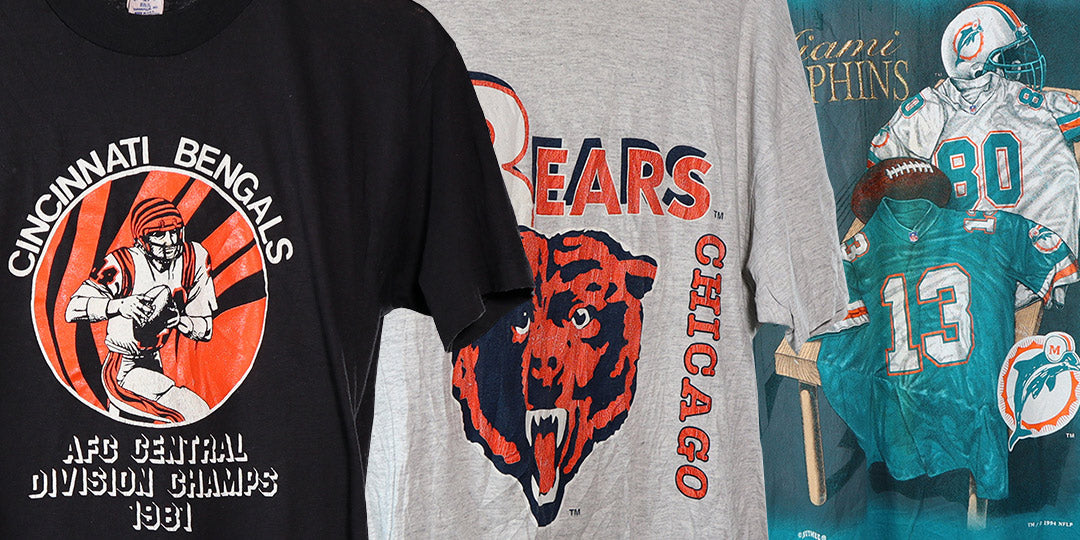The photograph showcases a display of sports-themed t-shirts and a poster. On the leftmost side is a black t-shirt featuring a design of an American football player. Around the player, the text reads "Cincinnati Bengals AFC Central Division Champs 1981." Partially obscured by the black shirt, the middle t-shirt is light gray and features an orange and black face of either a lion or a bear, with the words "Bears Chicago" around the image. On the right side of the image, there is a poster with a blue and white color theme. The poster displays various sports t-shirts, an American football, and a helmet, indicating that these items are likely part of a sports memorabilia display.